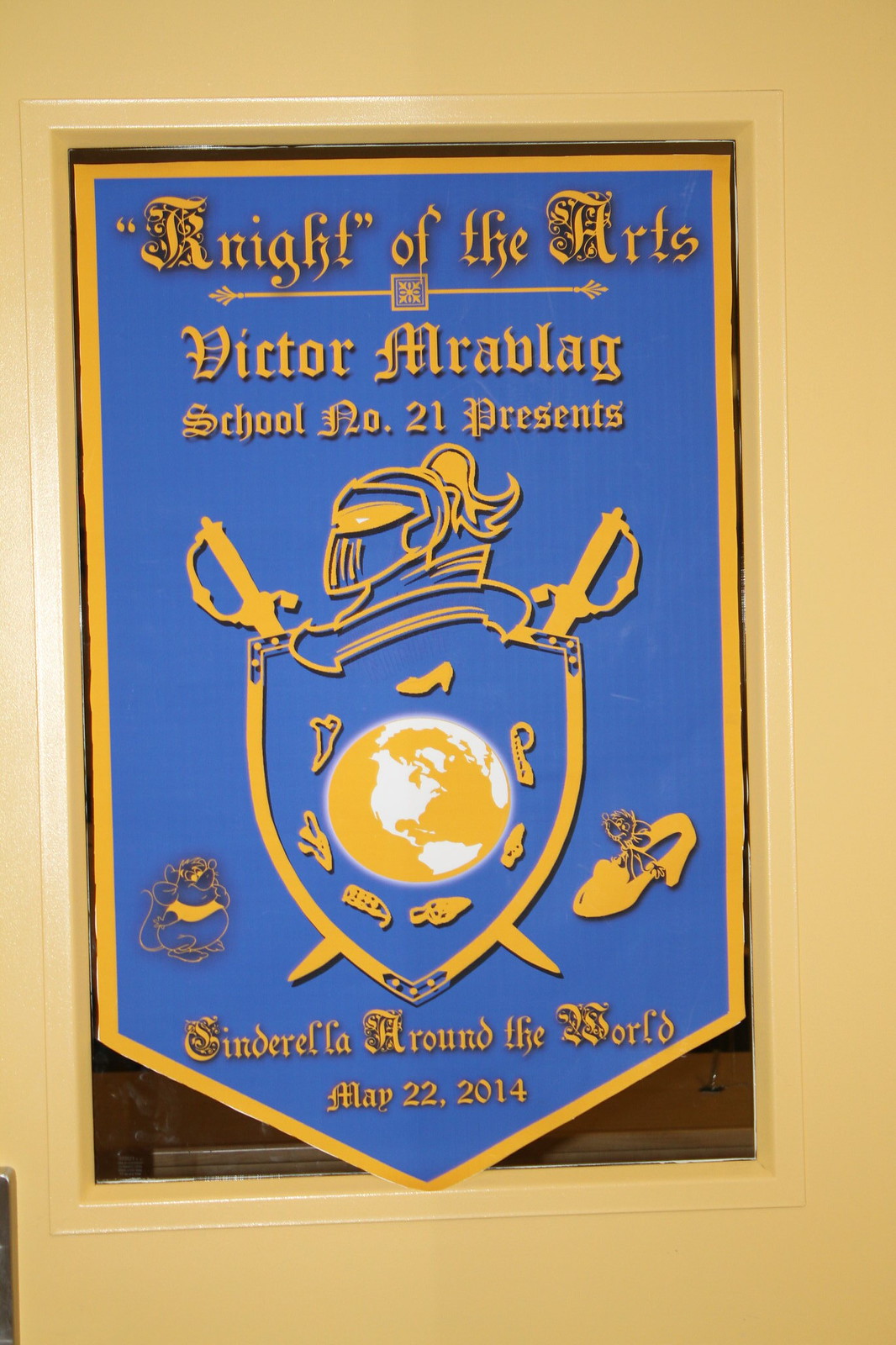This image shows a flag displayed in a tall rectangular window, which is slightly tilted to the left within a yellowish-tan metal wall, possibly a door. The flag features a unique design with straight 90-degree angles at the top and a downward-pointing triangle bottom. It has a thick yellowish-orange border and a bright blue background. The flag contains elegant yellow text saying, "Knight of the Arts, Victor Mrablag, School Number 21 Presents, Cinderella Around the World, May 22, 2014." Central to the flag is a detailed insignia depicting a shield with a globe, accompanied by various objects including shoes, which resemble slippers, and other small illustrations possibly depicting animals like mice. The illustration is adorned with the head of a knight and the hilts of swords branching out from the shield.